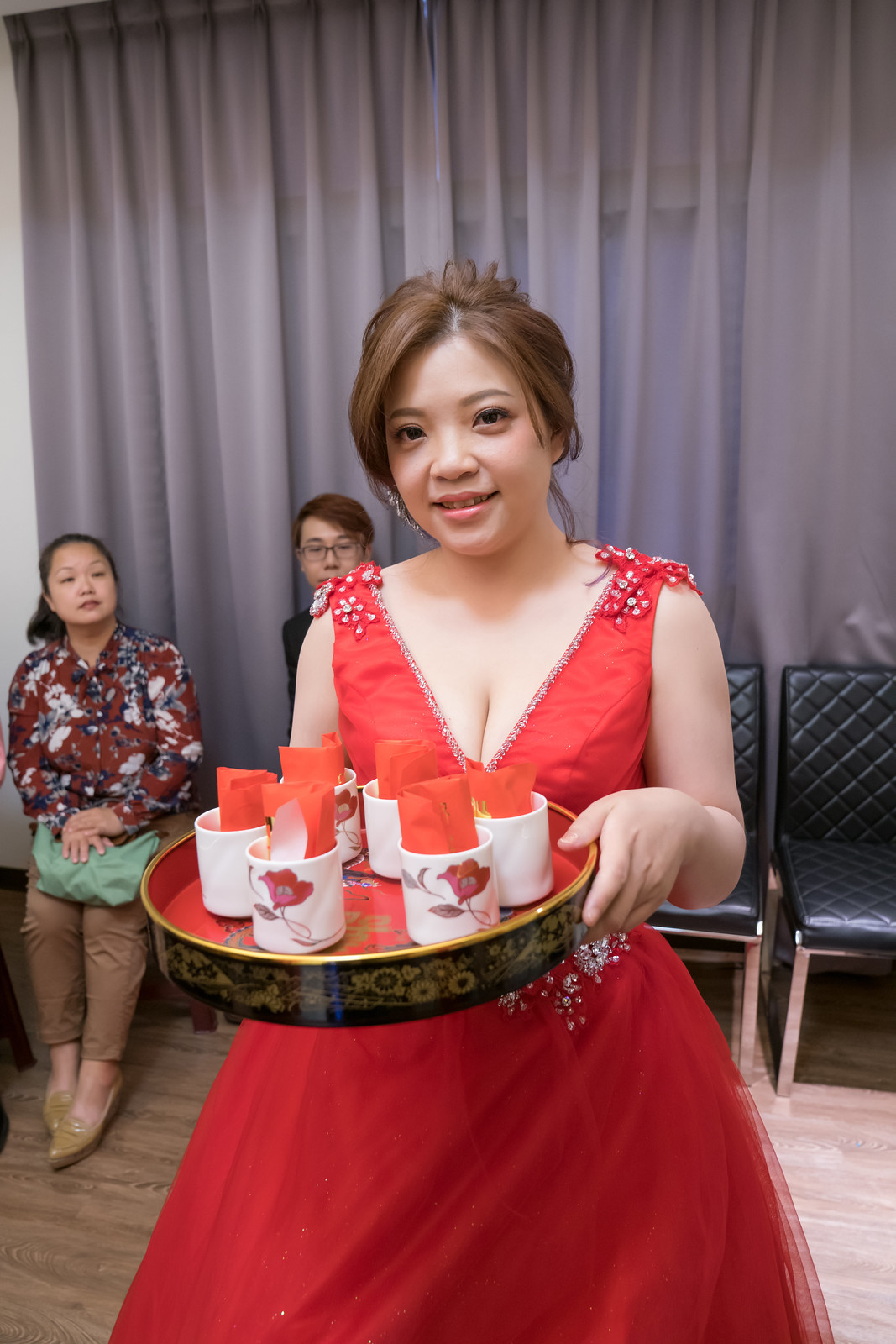This indoor photograph features a woman of Asian descent standing in the foreground, who is the focal point of the image. She has medium to light brown hair and is wearing a simple yet elegant red dress. She is smiling warmly and holding a decorative tray adorned with golden designs around its circumference. The tray contains mugs with floral designs and red papers inside them.

In the background, there's a tall, wide, somewhat transparent grayish-purple curtain that appears to either cover a window or serve as a room divider. Seated to the left is another woman of Asian descent, wearing brown pants, a deep red floral shirt, and pointy-toed shoes, with a mint green bag resting in her lap. Approximately a foot to her right is a man with short brown hair and glasses, who remains partially obscured. The woman is seated on a chair, while the man seems to be on a different, possibly black, chair.